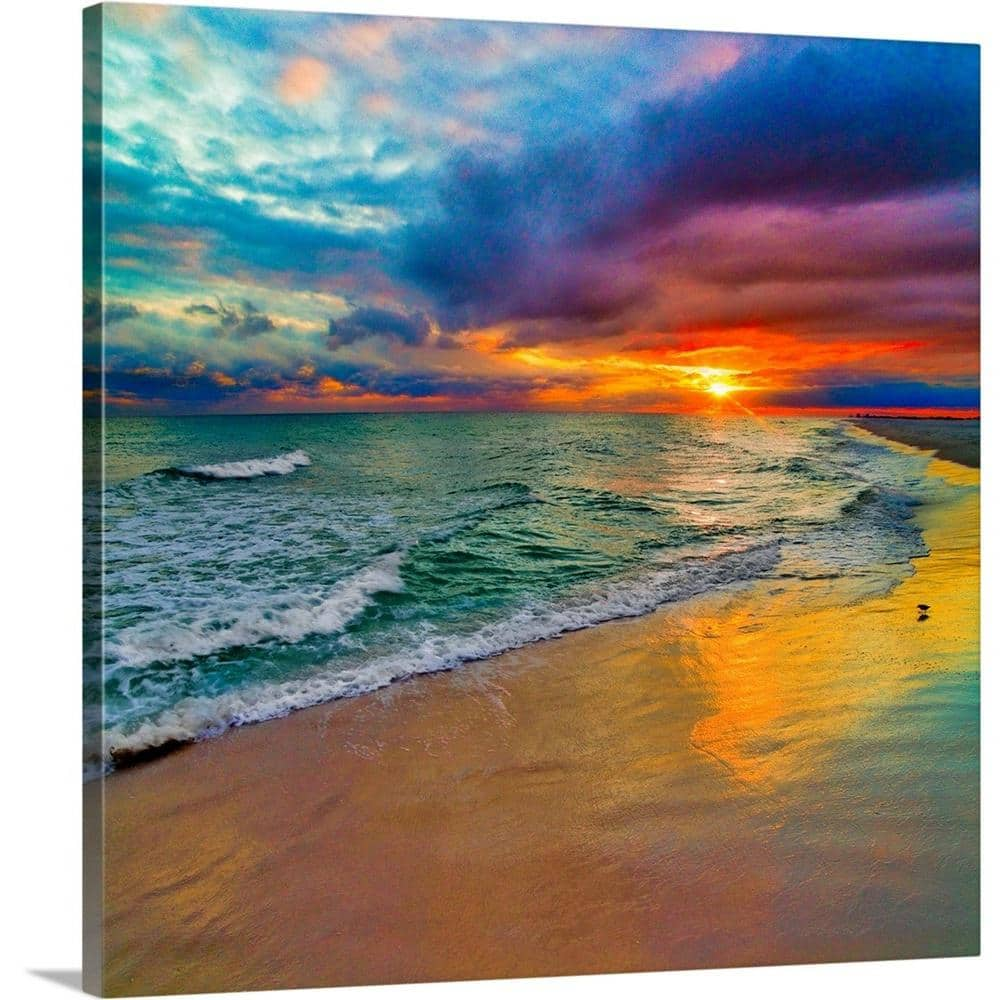The image is a vibrant, colorful art print of an ocean scene at sunset, captured on a canvas that's slightly tilted to the right, revealing its edge where the artwork continues. The scene depicts waves curling and foaming as they reach the yellow-hued sand, reflecting the sunlight. A tiny, indistinct bird sits on the shore, gazing at the approaching waves. The ocean water is a light green, while the sky is a breathtaking blend of purples, blues, and golds. The sun setting on the horizon casts a reddish-yellow glow, contrasting with the dark blue and purple clouds overhead. As the sky clears toward the left, more blue sky becomes visible. The clouds, in various vibrant shades, reflect the brilliant colors of the sunset, creating a stunning display that cascades down to the sand, which mirrors these warm golden, amber, blue, purple, and green hues from the horizon to the foreground.